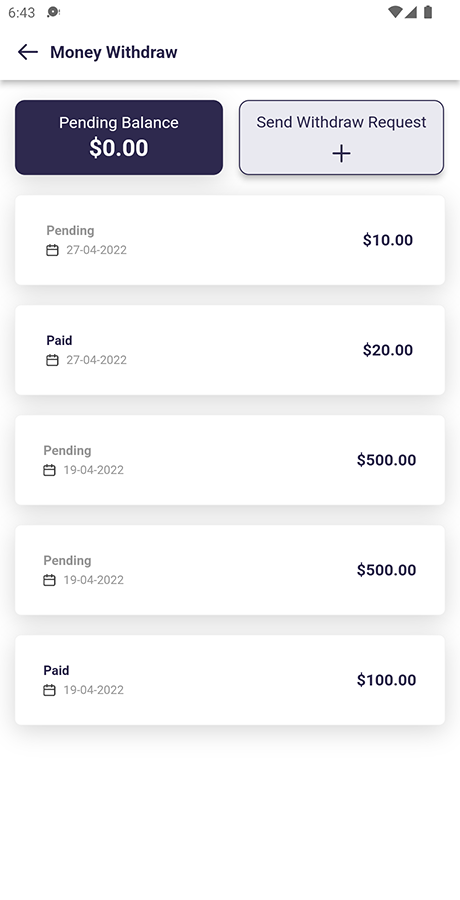A detailed image description of a smartphone screenshot capturing a financial app interface, possibly similar to PayPal:

At the top of the screen, the status bar displays the current time on the left, showing "6:43" alongside a circle icon that likely represents a memory function. On the right side of the status bar, fully filled icons for Wi-Fi, data, and battery are visible, all displayed in dark gray text.

Below the status bar, there's a header section in dark blue text indicating "Money Withdraw," accompanied by a back arrow icon on a white background. This header is separated from the rest of the content by a gray dividing line.

The next section features text in white against a blue background, stating "Pending Balance: $0.00." Adjacent to this, a button with a blue outline and light blue background reads "Send Withdraw Request," marked by a plus symbol.

Beneath this interface, a series of rows list various transaction requests, either pending or paid. Each row includes the status of the transaction—either "Pending" or "Paid"—followed by the date and amount. Additionally, a calendar icon appears below the status in each row.

The specific transactions listed are as follows:
- Pending, 27-04-22, $10
- Paid, 27-04-22, $20
- Pending, 19-04-22, $500
- Pending, 19-04-22, $500 (appears twice)
- Paid, 19-04-22, $100

These transactions fill up the lower portion of the screen, detailing the various payment statuses and amounts associated with each date.